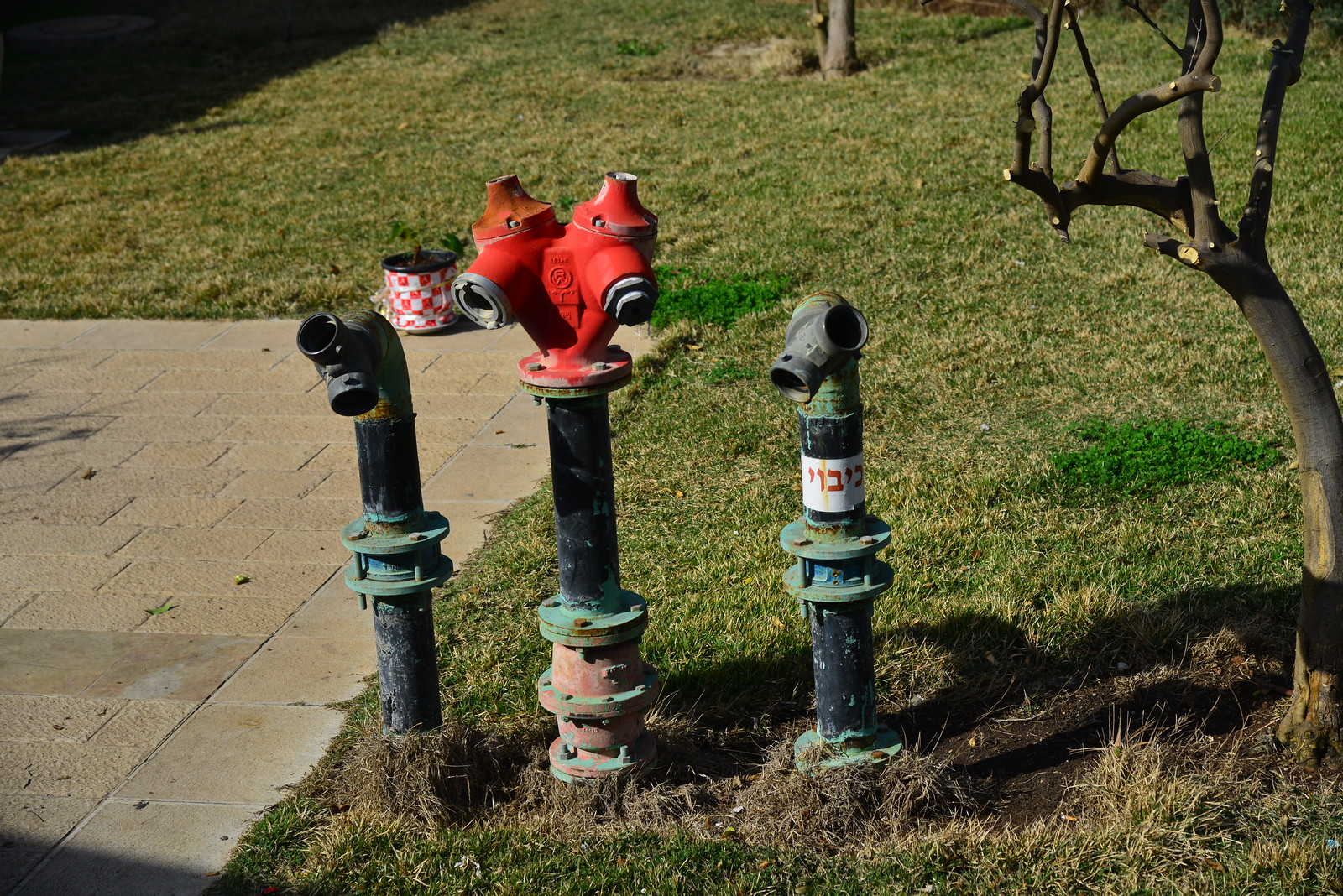In the foreground of the image, three metallic pipes, possibly fire hydrants or water access points, extend from a grassy field. The pipes are predominantly dark in color, with the left and right pipes each having two openings; one points inward and down, the other outward and up. The middle pipe, which is brown at the base with a red cap on top, features two valves extending from the left and the right. All three pipes have bolted sections visible, particularly the green segments.

Surrounding the pipes, the grass looks recently mowed, interspersed with patches of clover or similar plants. To the right, there is a small, recently trimmed tree. In the distant background, the trunk of another tree is visible. A stone-paved area occupies the bottom left corner, and to the left of the image, a patterned sidewalk made of bricks runs downward. On this walkway, a plant in a pot adorned with red and white patterns is just beginning to grow.